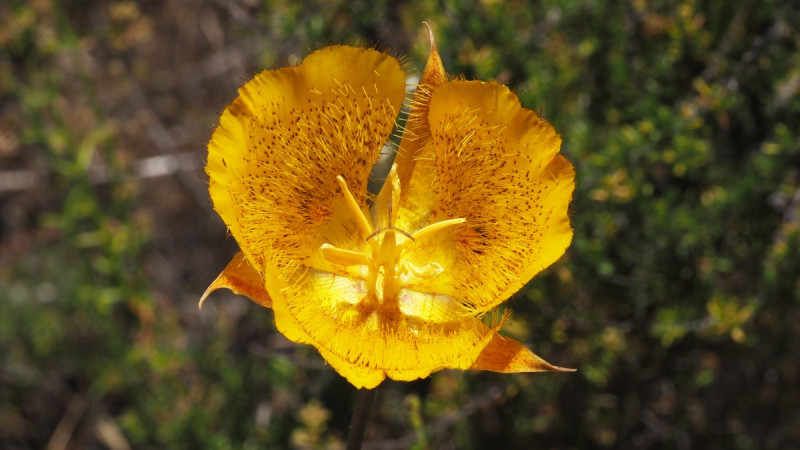This close-up photograph captures a detailed and vibrant yellow flower with brown speckles and striping. The flower's two large upper petals are intricately speckled with an orangey-brown color, and their edges are rimmed with fine, yellow hair-like fibers that catch the light, making them appear shiny and reflective. At the flower's center, several distinct yellow threads, resembling hair-like appendages, radiate outward. The background of the image is artistically out of focus, featuring a blend of green, brown, and yellow foliage, alongside some white and brownish twigs, which enhances the flower's prominence as the photo's main focal point.